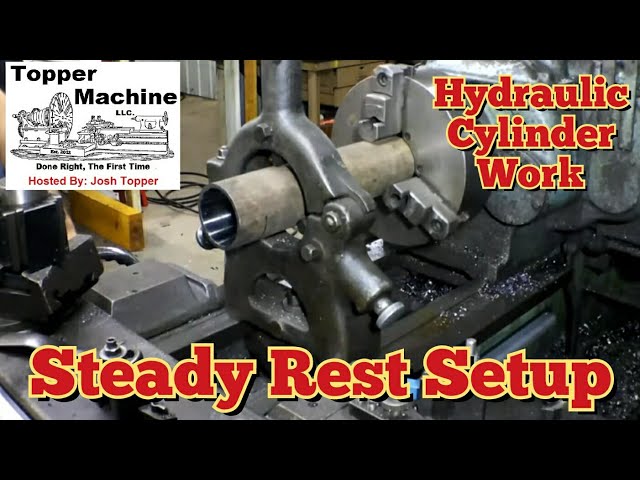The image shows a cylindrical machine prominently filling most of the frame, with a black strip along the top and bottom. The machine features a large cylindrical body on the right and a smaller cylindrical axis extending from the left end, encased in metal housing with arms extending upwards and downwards. It's positioned on an irregular gray tabletop surface surrounded by low-lying machinery and scattered metal shavings. In the upper right corner, bold red text with a yellow border reads “Hydraulic Cylinder Work,” while along the bottom, similarly styled text declares “Steady Rest Setup.” In the upper left corner, inside a white square, a black line diagram of machinery is labeled "Topper Machine," in reference to the headline "Done Right the First Time," hosted by Josh Topper.